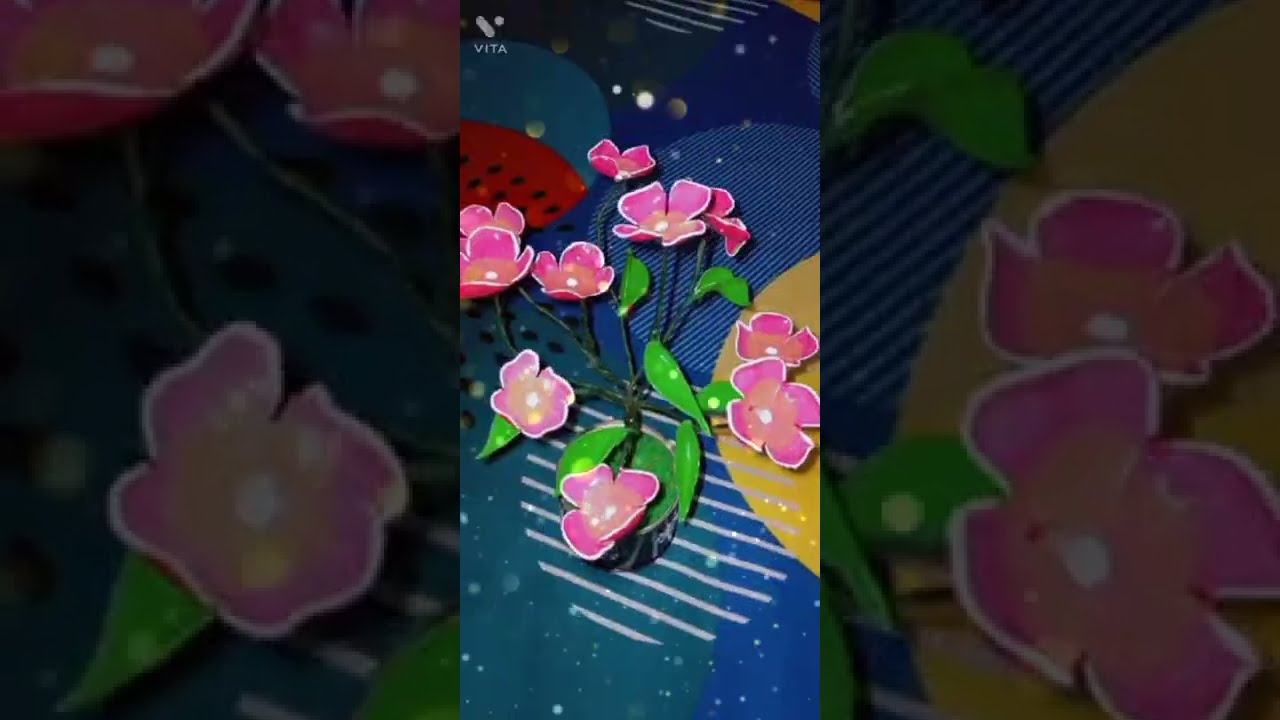In the center of this graphic art piece, there is a detailed depiction of artificial pink flowers with yellow centers, possibly made of fabric or another synthetic material. These flowers, surrounded by scattered green leaves, are situated on a predominantly blue background adorned with various shapes, including half-arcs, circles, and patches of different colors—yellow, red, and darker blue. The background fabric appears textured, reminiscent of denim, and it features white lines and spots. Positioned in the top left corner of this artwork, there is the word "VITA" written in bold white capital letters, accompanied by a stylized 'V' above the text, suggesting a branding or advertising element. Additionally, the image is divided into three panes, with the two side panes showing zoomed-in, darkened sections of the flower petals from the central panel, creating a picture-within-a-picture effect. This layered visual composition might evoke the whimsical feel of a child’s play area, further emphasized by the bright, vibrant colors and tactile elements.